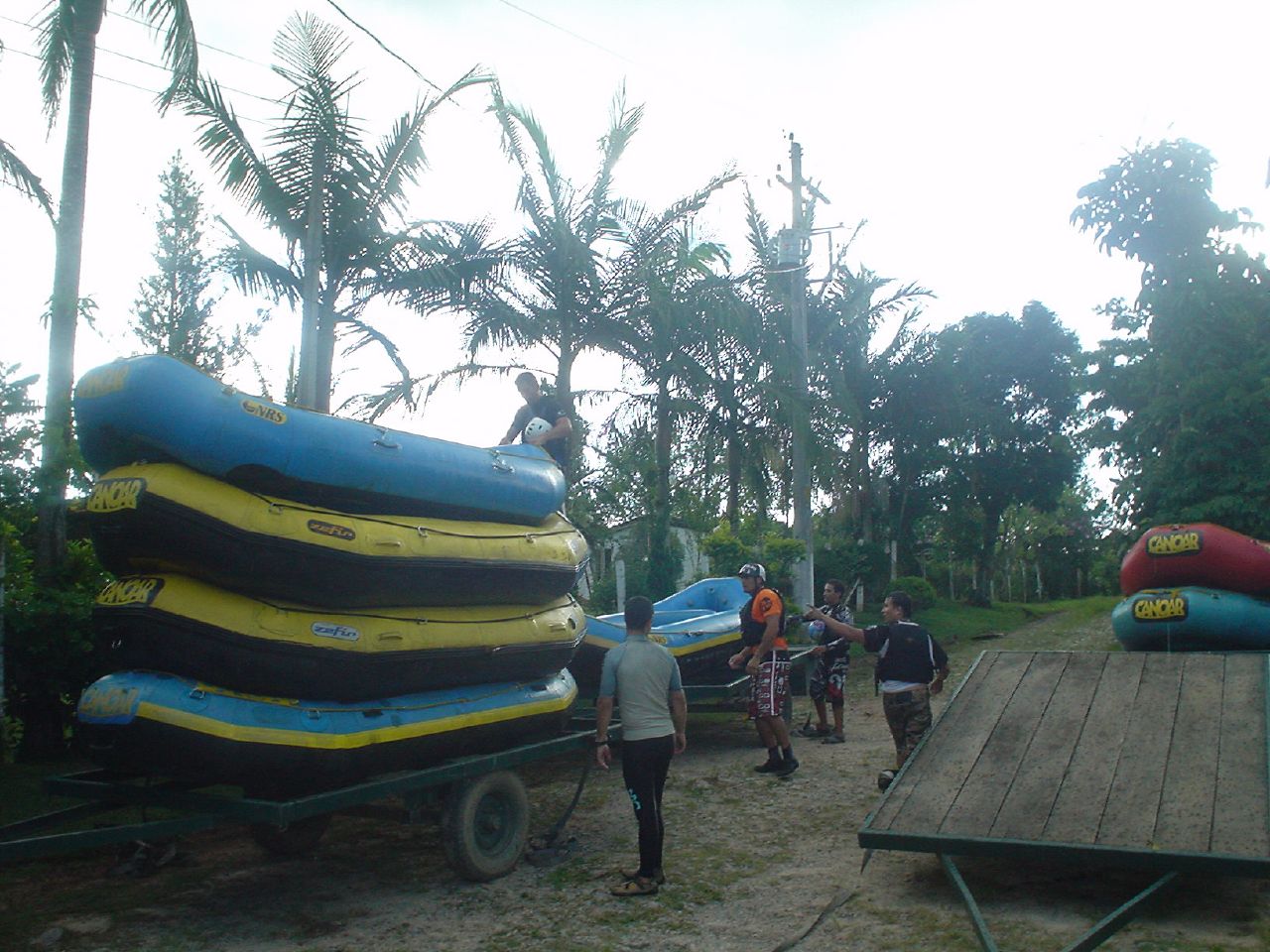The somewhat out-of-focus photograph captures an outdoor scene on a bright day, making the sky appear washed out. The setting is a dirt road with grassy patches and palm trees, as well as an electrical pole in the background. Central to the image are three trailers, each holding varying numbers of inflatable rafts typically used for river rafting trips. The trailer closest to the viewer has four stacked rafts—two blue and two yellow—with a man climbing to the top carrying a white helmet. A second trailer holds a single raft colored blue and black, and nearby, a third trailer with a wooden floor awaits loading, with two additional rafts at its side. Five people are present; one man on the ground wearing a helmet and life jacket, along with others mingling or helping with the rafting equipment. The lighting conditions obscure some details, but the overall busy and preparatory mood of the scene remains evident.